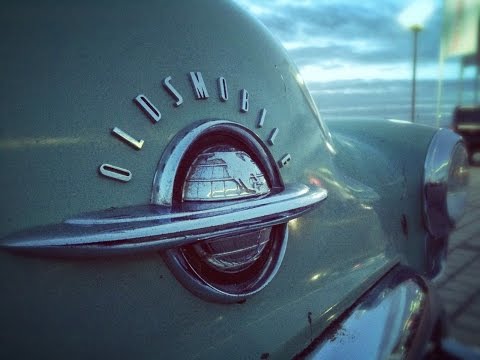In the image, there is an old, weathered Oldsmobile prominently featuring the front hood. The car has a dull, flat gray color and is adorned with chrome accents. On the right side, a round headlight is visible. The centerpiece of the hood showcases the Oldsmobile logo: silver letters curving around a globe with continents and grid marks, crossed by a silver chrome line. The car appears to be parked on bricks, suggesting it might be stationary for a long period. The background reveals a cloudy sky with hints of light, potentially signaling sunrise or sunset, and a body of water, likely an ocean. Additionally, a lit lamp or streetlight and some sort of wooden structure can be seen to the right, contributing to the overall gray and somber atmosphere of the scene.